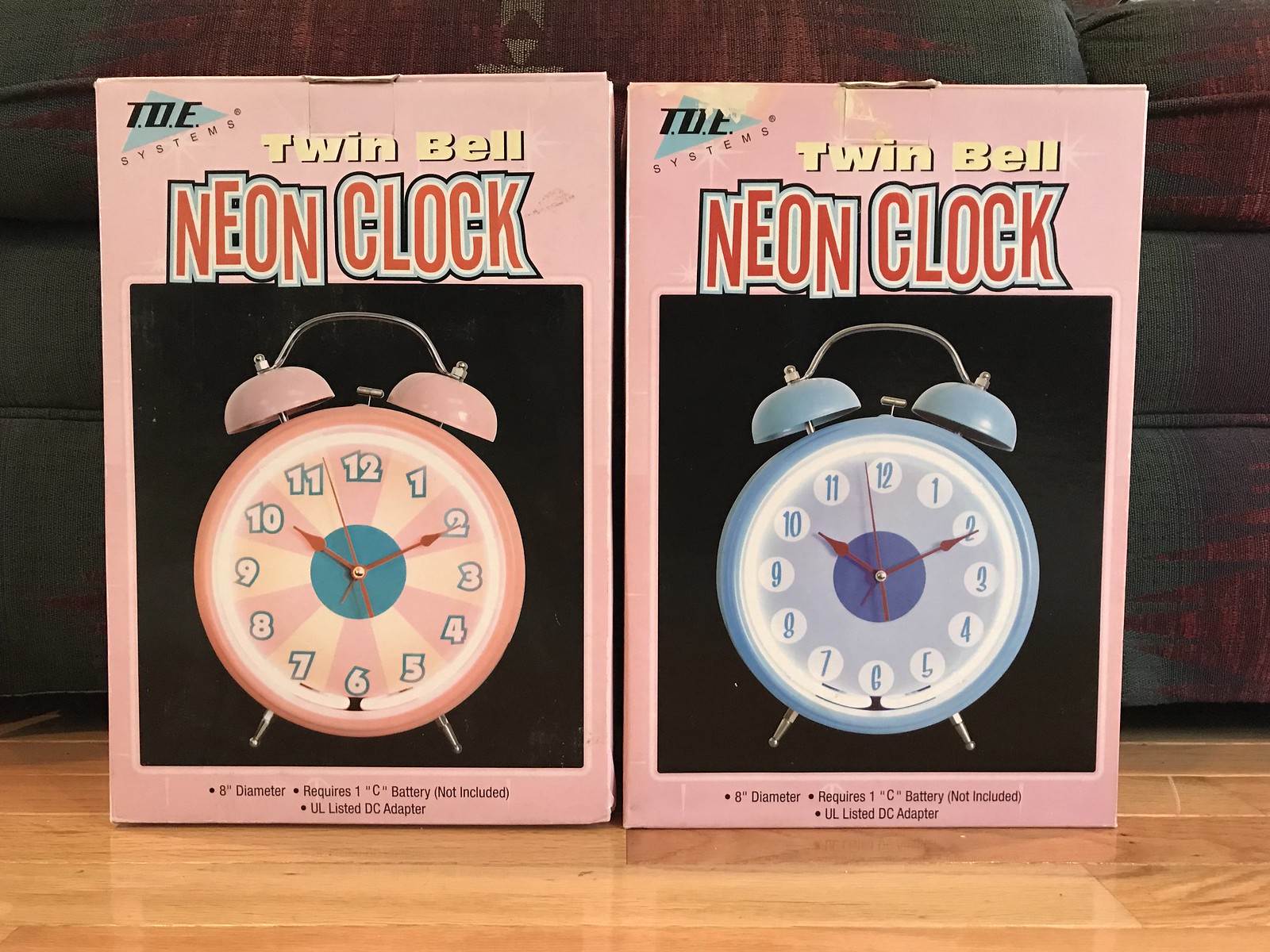This vibrant photograph features two vertically rectangular, retro-style boxes positioned side by side on a shiny wood grain living room floor with a fluffy, overstuffed, dark bluish-gray couch in the background. Each pink box prominently displays the text "TDE Systems Twin Bell Neon Clock" at the top. A large black square in the center of the box showcases the vintage clock inside. The box on the left shows a pink clock with matching pink bells and a pink frame, accompanied by large white block numbers and red hour and second hands. The box on the right features a blue clock with similar design elements, including blue bells, a blue frame, and red hands. Below the clock image, additional details read "8-inch diameter, requires one C battery not included, UL listed, DC adapter." The overall scene exudes a nostalgic charm, further enhanced by the light casting gentle shadows on the wood grain floor, emphasizing the retro appeal of these Twin Bell Neon Clocks.